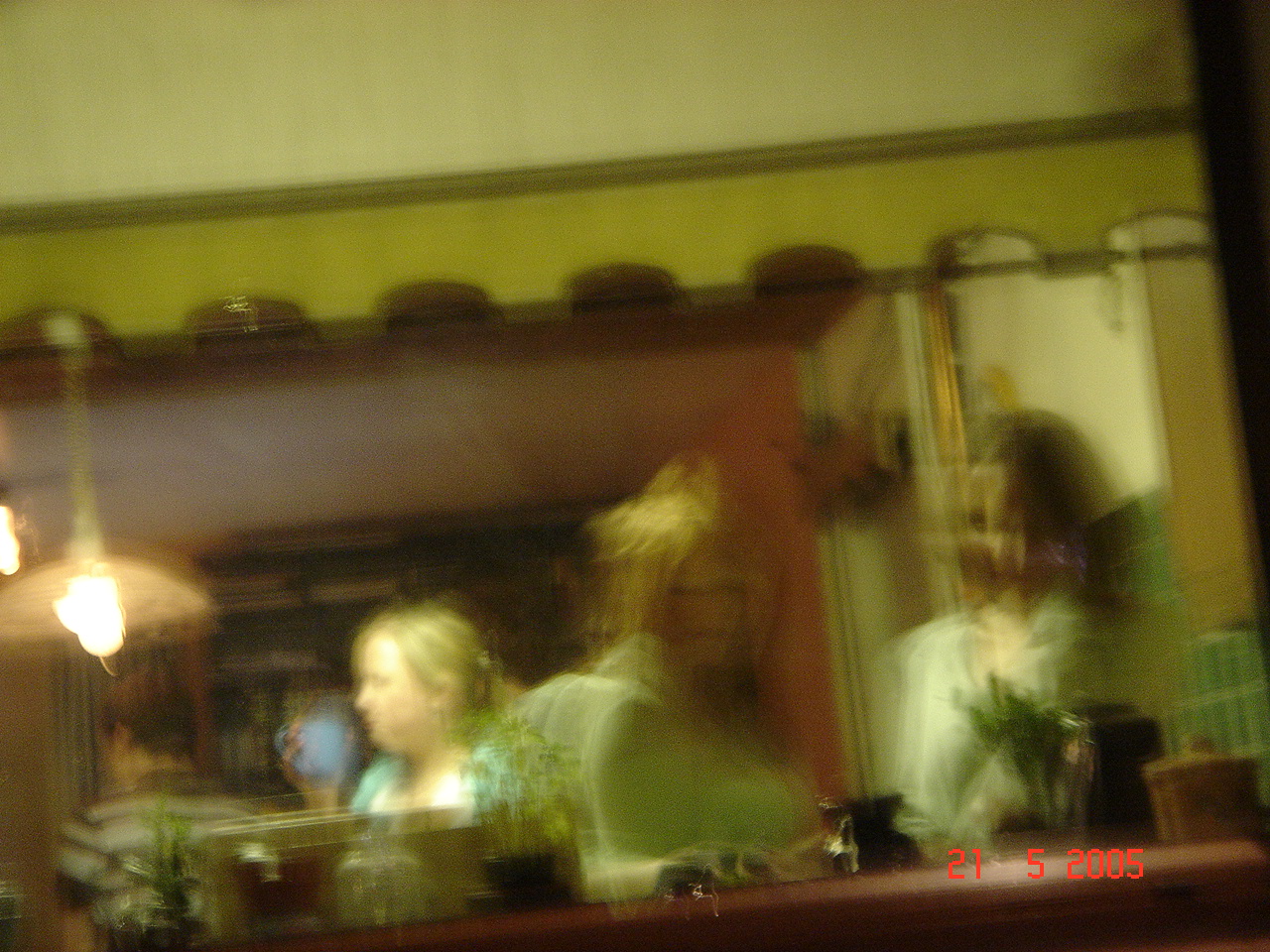This extremely blurry photograph, likely taken with a digital camera on May 21st, 2005, captures a kitchen-dining area in a residential home, distorted due to camera movement. It features three women engaged in conversation and activities around what seems to be a dining table or breakfast bar, as indicated by a low-hanging lamp with a chain. One woman, with blonde hair pinned up with a hair clip, holds a blue coffee cup. Another woman with dark hair wears a white top, and a redheaded woman, also in white, stands nearby. Observably, the kitchen has a high ceiling, with a complex background including a large wooden cabinet or possibly a fireplace, segmented in dark brown. On the right, a rack, perhaps a napkin holder, is visible on a table. The setting includes additional details like flowers on a countertop and a shelf or display area featuring dishware. Another individual in a brown and white striped shirt with short brown hair appears almost at the bottom left corner, partially visible through the reflection in a mirror with a scalloped top edge. Draped windows and divider walls suggest a typical home dining environment, adding depth to the scene.